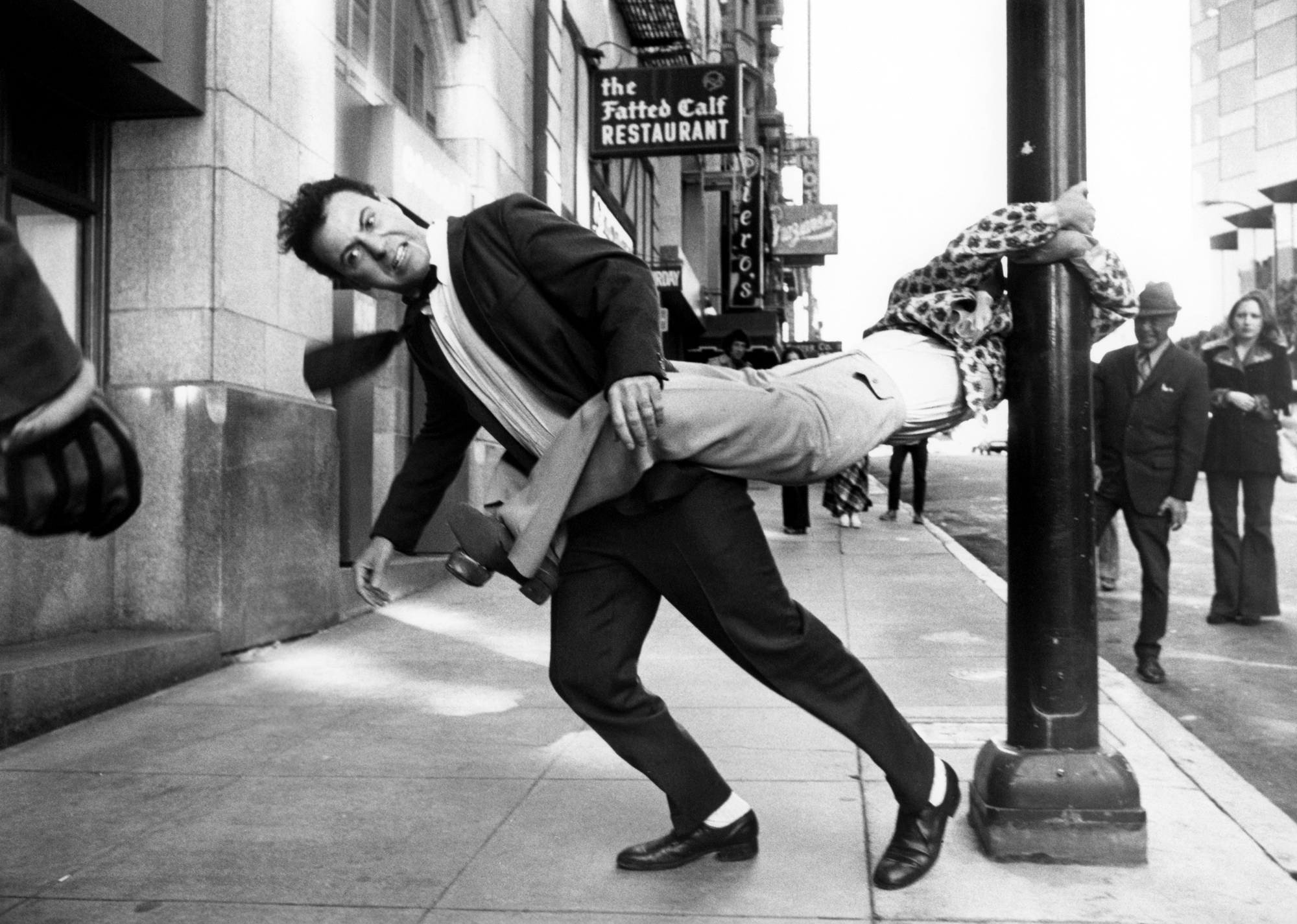This humorous black-and-white photograph captures a bustling city sidewalk scene. Dominating the center, a man in a polka-dotted coat with khaki pants is comically wrapped around a street lamp pole, his arms and legs clinging tightly. His legs are also wrapped around another man who appears to be struggling to escape. This second man, dressed in a dark suit, black pants, white socks, and black shoes, is leaning forward with a grimace on his face, his tie flying as he braces himself against the pull. Both men draw attention from passersby, with some smiling or laughing at the spectacle. In the background, a sign reading "The Fatted Calf Restaurant" is prominently displayed on a building, adding context to the urban setting. Further down the street, another sign appears to read "Peros.” The scene exudes a lively and chaotic energy, enhanced by the people in the background, including a man in a suit and hat laughing, and a woman in dark bell-bottom pants. This photograph not only captures an amusing moment but also the vibrant life of a busy city street.